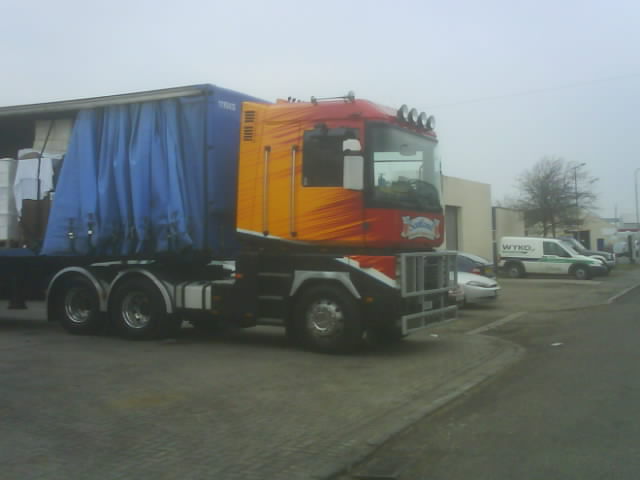This square, full-color photograph captures an overcast, somewhat misty day in an industrial park, characterized by grayish-blue skies. In the background, small low commercial buildings with vans and cars parked beside them are visible. Dominating the foreground is a vibrant, semi-truck. The cab, adorned with an orangey-red and yellow fire paint design, features a large 8-10 foot windshield and a light bar up top. The truck’s large doors suggest its role in transporting substantial items. The trailer, partially open, reveals blue canvas curtains and various large tubs or reams of paper secured inside, indicating the vehicle is likely used for delivering sizable objects.